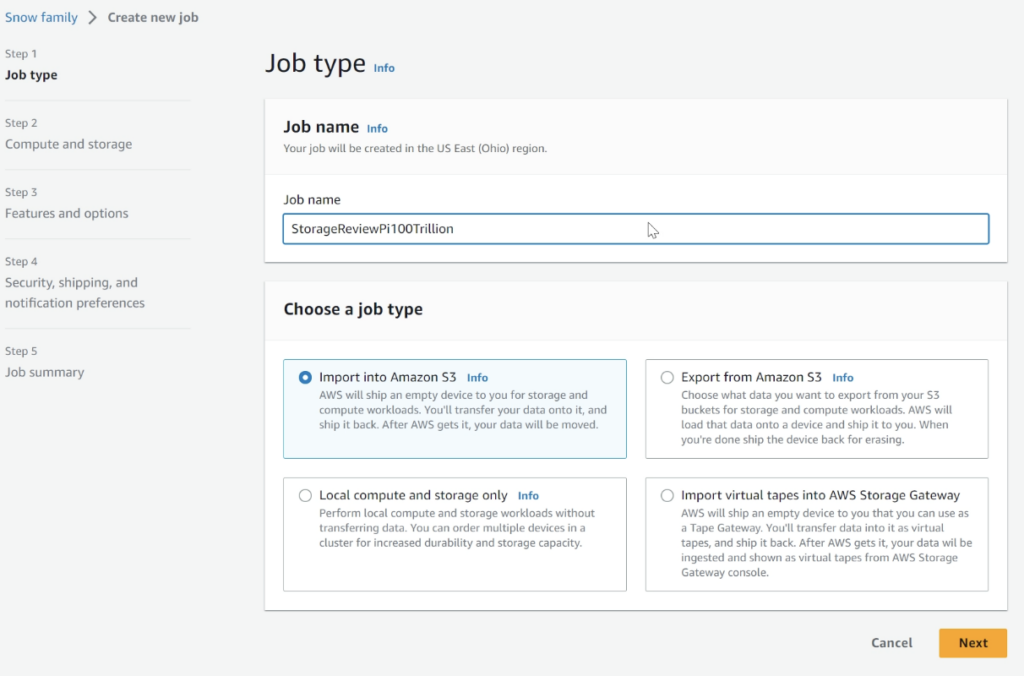The website displayed on the computer screen is divided into two sections, with the left-hand side being smaller. On the left, the words "Snow Family" are highlighted in blue, followed by a series of steps detailing the sequential process of creating a job:

1. **Step 1: Job Type**
2. **Step 2: Compute and Storage**
3. **Step 3: Features and Options**
4. **Step 4: Security, Shipping, and Notification Preferences**
5. **Step 5: Job Summary**

Each step is separated by a horizontal line. 

Towards the center of the screen, under the "Job Type" section, there is an "Info" button in blue and a large triangle symbol. Below, the text "Your job will be created in the U.S. East (Ohio) region" is prominently displayed. 

The "Job Name" field is accompanied by another "Info" button in blue. Below this, there is a long, thin blue rectangle labeled "Storage Review" showing "P100 Trillion." 

Further down, a selection box presents four job type options:

1. **Import to Amazon S3**
2. **Export from Amazon S3**
3. **Local Compute and Storage Only**
4. **Import Virtual Tapes into AWS Storage Gateway**

The screen indicates that the first option, "Import to Amazon S3," is currently selected.